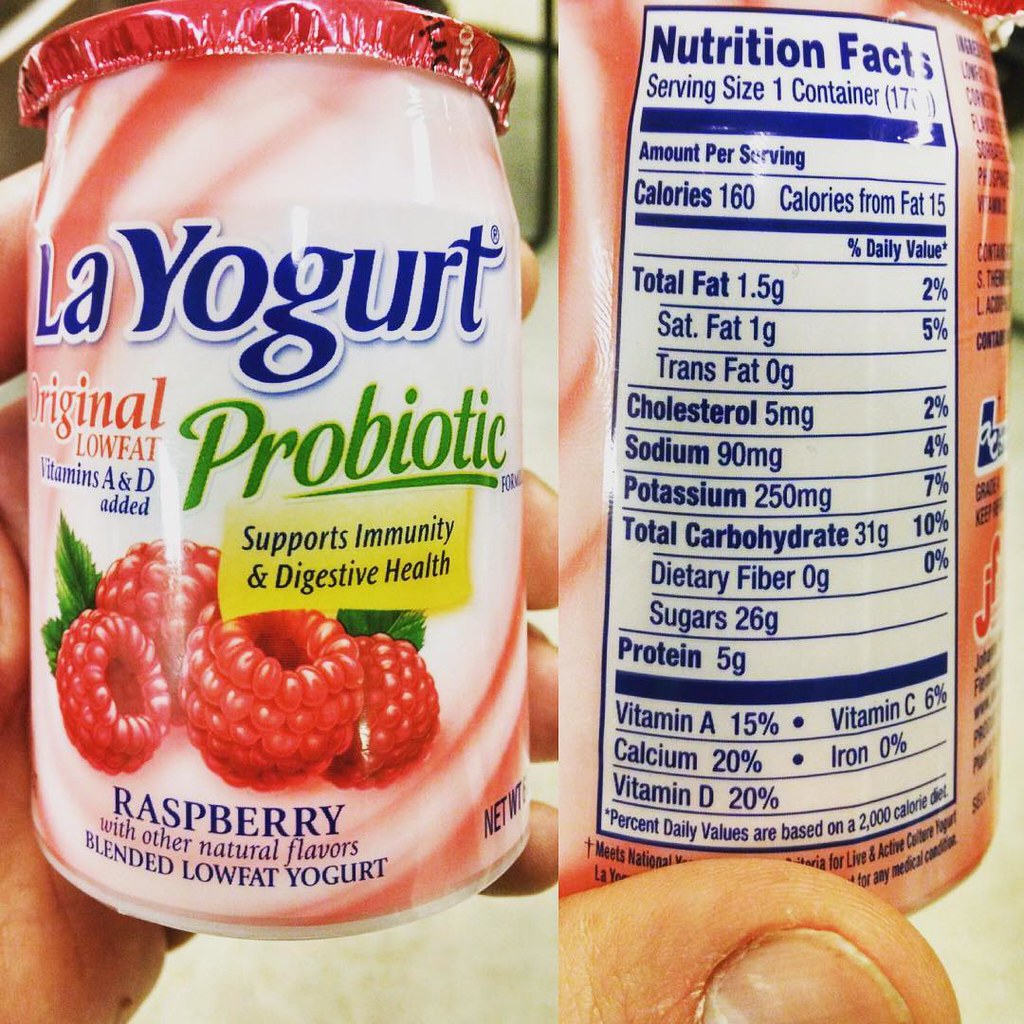The image features a split photograph of a yogurt product called "La Yogurt." The left side of the picture showcases the front of the product. It has a distinctive pink lid and a visually appealing white and pink spiral-striped label. The brand name "La Yogurt" is prominently displayed in bold blue letters with a white outline. Below the brand name, in red letters, it states "Original Low Fat." Further details include blue text indicating "Vitamins A and D Added" and green text for "Probiotic." A blue banner highlights that the yogurt supports immunity and digestive health, while a yellow banner with blue letters reiterates this claim.

The label also features vibrant images of raspberries along with the flavor description "Raspberry" in blue letters. It is noted that the yogurt is a "Blended Low Fat Yogurt with Other Natural Flavors."

On the right side of the photograph, the nutritional facts are laid out against a white background in blue letters. Key nutritional information includes:

- Serving Size: One container
- Calories: 160 (15 from fat)
- Total Fat: 1.5 g (Saturated Fat: 1 g, Trans Fat: 0 g)
- Cholesterol: 5 mg
- Sodium: 90 mg
- Potassium: 250 mg
- Total Carbohydrate: 31 g (Dietary Fiber: 0 g, Sugars: 26 g)
- Protein: 5 g

A prominent thick blue line separates the macronutrient information from the vitamin content, which details:
- Vitamin A: 15%
- Calcium: 20%
- Vitamin D: 20%
- Iron: 0%
- Vitamin C: 6%

This detailed and colorful packaging highlights both the product features and nutritional information, making it easy to identify and understand the health benefits of this yogurt.